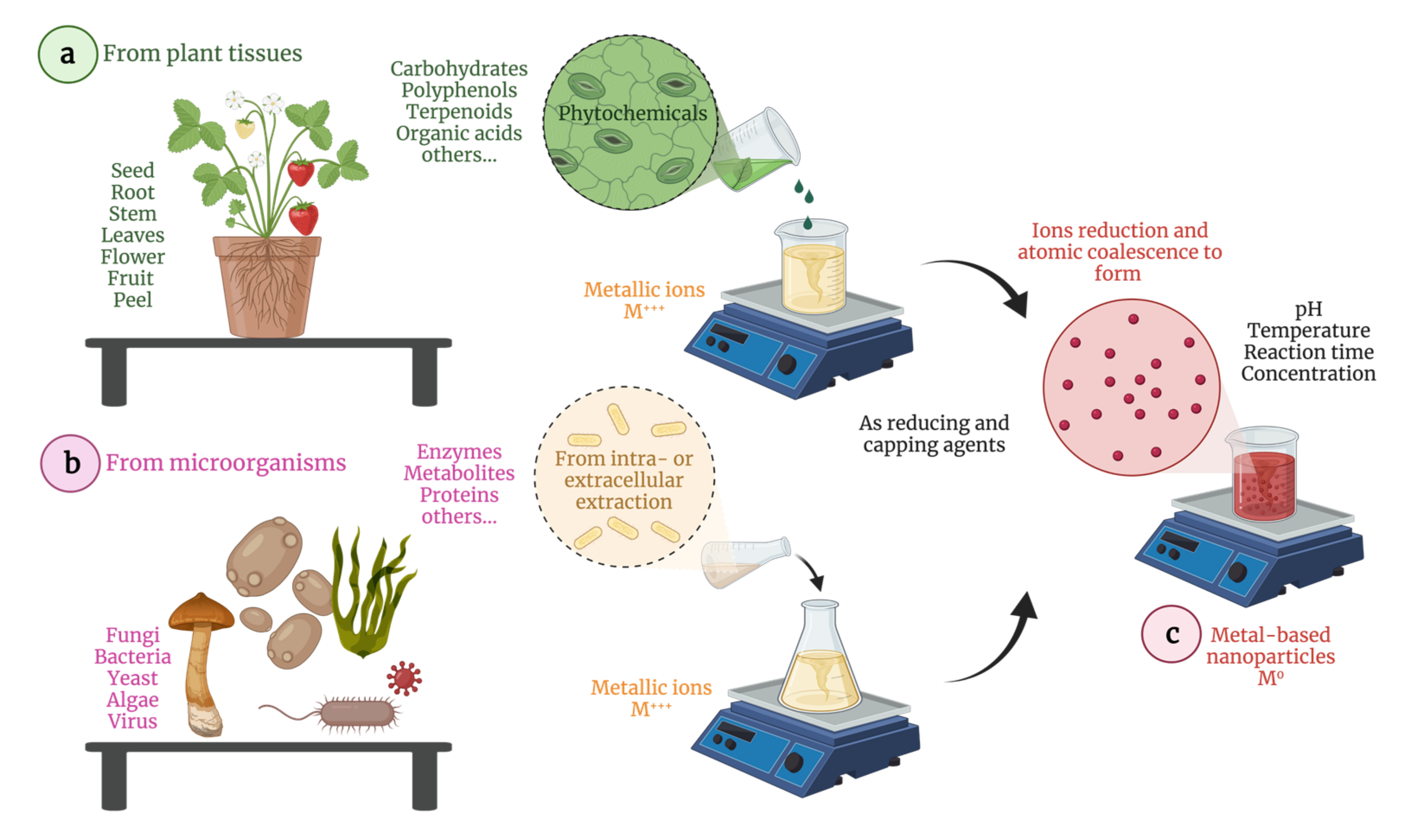This detailed diagram showcases the process of converting plant tissues and microorganisms into metal-based nanoparticles. On the left side, under a green heading that reads "From Plant Tissues," a flower pot is depicted on a small stand containing a strawberry plant, with labels pointing to different parts of the plant: seed, root, stem, leaves, flower, fruit, and peel. Next to the plant, illustrations of various microorganisms—fungi, bacteria, yeast, algae, and virus—are included.

To the right of these elements, there is a series of scales and beakers filled with liquids, accompanied by annotations like "Photochemicals from intracellular or extracellular extraction" and "reducing and capping agents." One of these beakers, filled with red liquid, is situated on a smaller scale. Additional text includes terms such as "photochemicals, carbohydrates, polyphenols, terphenols, organic acids, others" which drip into another beaker containing tan liquid labeled "metallic ions, M." An arrow points from this beaker to another circle indicating the process of "ions reduction and atomic coalescence to form metal-based nanoparticles."

The entire diagram is colorful and illustrated in a clip-art style, set against a white background, with a general lack of detailed explanations, making it appear more understandable to those already familiar with the topic.